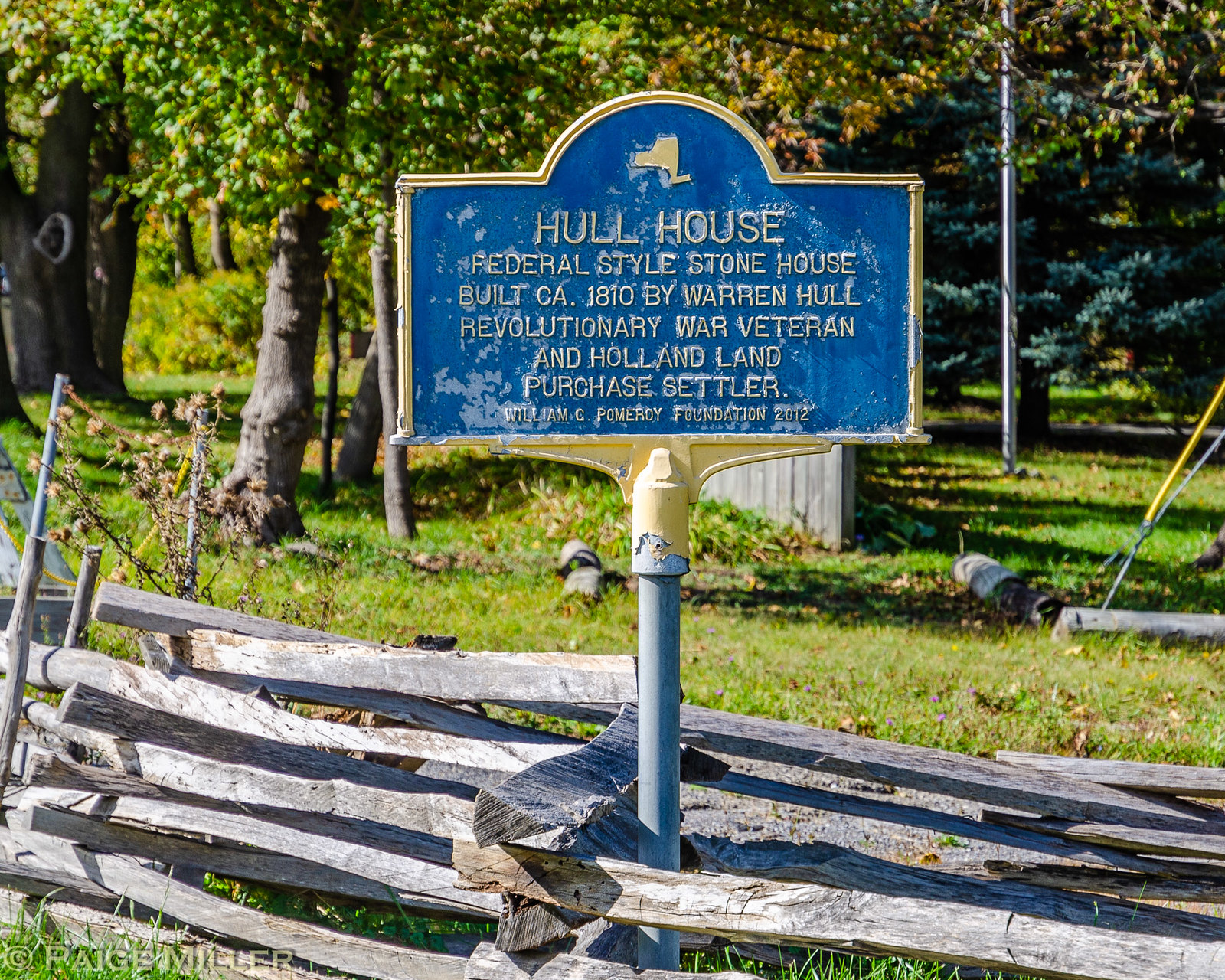In a serene grassy field area, an aged historical sign marks its presence, firmly entrenched in the soil on a sturdy metal pole. This blue rectangular sign, topped with a semicircular disc, is slightly weathered with flecks of blue paint chipped off, giving it a timeworn charm. Gold raised letters spell out the historical significance: "Hull House, Federal-style stone house, built C.A. 1810 by Warren Hull, Revolutionary War veteran and Holland land-purchase settler. William C. Pomeroy Foundation, 2012."

The sign is nestled between the rails of an old farm-style wooden fence, roughly three feet tall, which adds to the rustic ambiance of the scene. In the background, the vivid greens of the trees are accented by the gentle onset of autumn; leaves are starting to turn yellow and some have already carpeted the ground. Further back, approximately a hundred feet away, a flagpole stands, though only its base is visible in the image. This picturesque setting juxtaposes history with the quiet beauty of nature.